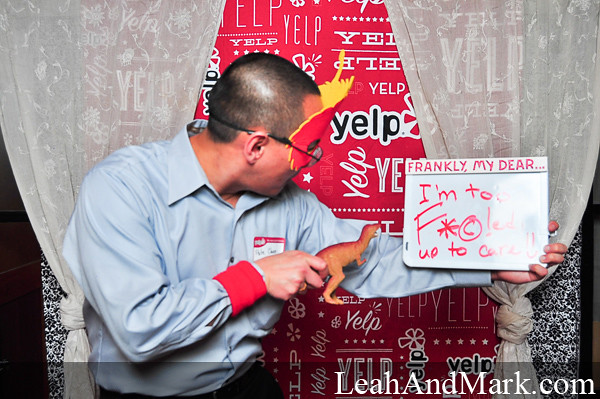A detailed image description: In front of a large red banner plastered with multiple Yelp logos and flanked by sheer white curtains, a man stands turned away from the camera. He is dressed in a light blue button-up shirt with a name tag featuring the Yelp logo in the top right corner. The man wears a striking red and yellow mask over his face, adding an element of playfulness and intrigue. In one hand, he holds a small toy dinosaur, while in the other, he displays a whiteboard. The whiteboard's message starts boldly at the top in red letters: "Frankly, my dear, ..." but becomes partially obscured by glare. It reads, "I'm too F***ing ... to care!" with various symbols filling in the expletive. At the bottom of the whiteboard, the text "leahandmark.com" is clearly visible, adding a touch of whimsy and curiosity to the scene.